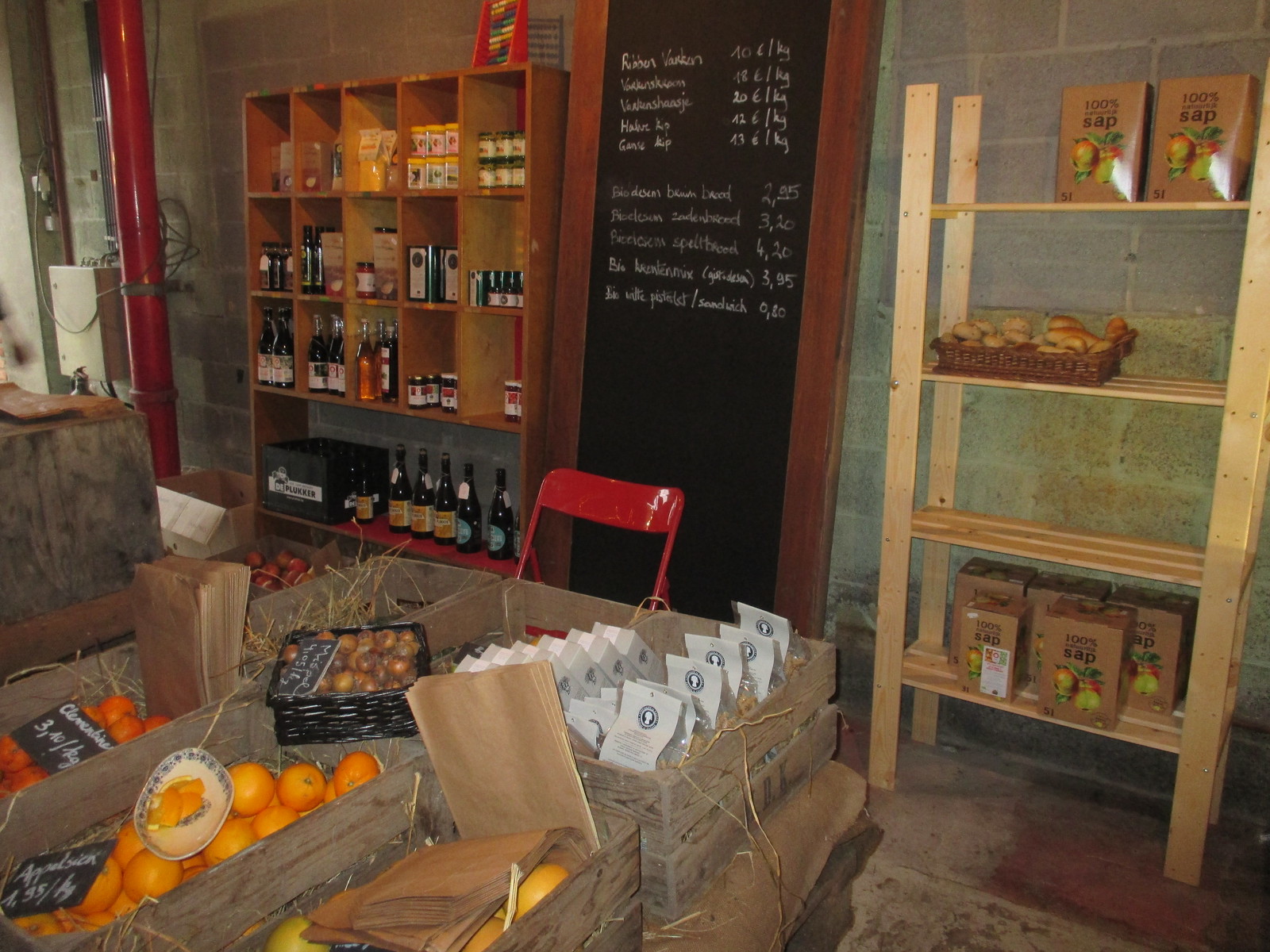The image depicts a scene inside a grocery store. Centered on a gray wall is a prominent black chalkboard with prices written on it in white chalk, advertising items that are difficult to read due to their small font. To the left of the chalkboard stands a wooden shelf with five columns and three rows, filled with an array of bottles, which could be wines or assorted jars. To the right of the chalkboard is another wooden shelf holding several brown bags. Small crates are visible in the foreground; some contain oranges, while others hold grapefruits. Above the fruit section, a sign reads "100% SAP." The detailed assortment and layout suggest the store specializes in diverse goods, including beverages, fruits, and possibly other gourmet items.